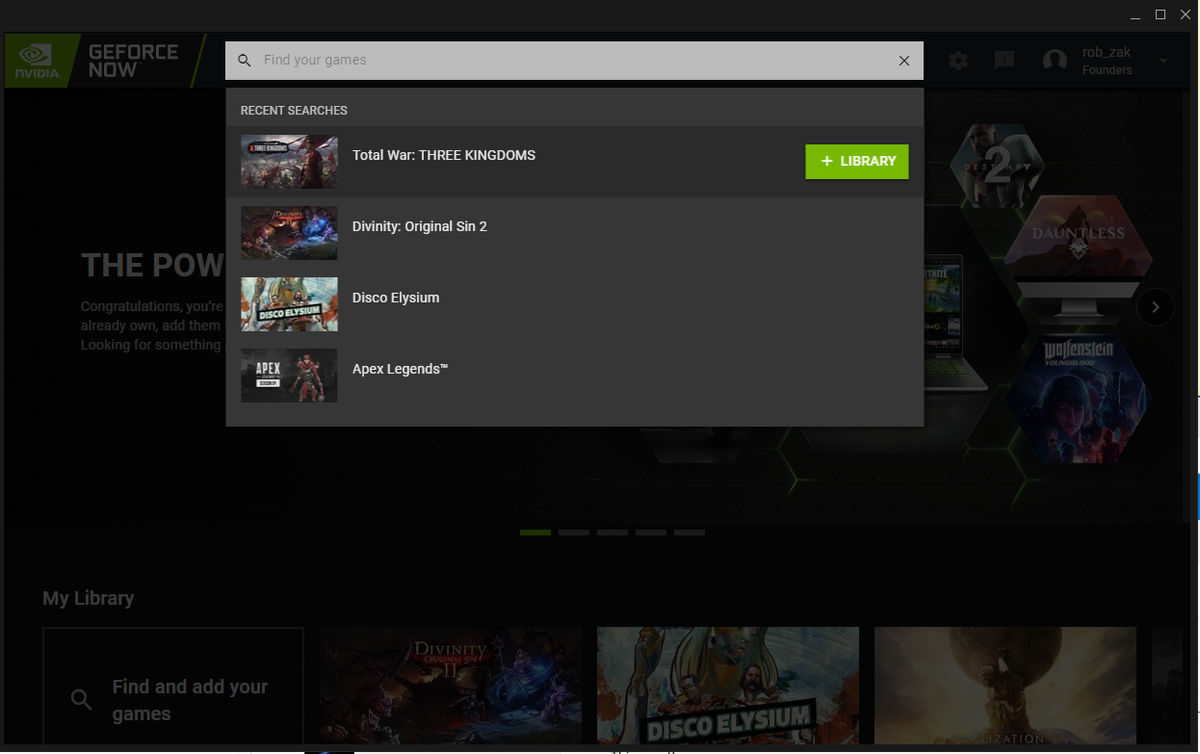Screenshot of the GeForce Now application interface:

The screenshot captures the GeForce Now app interface, which is designed to accompany the NVIDIA GeForce video card. The entire background has a black, darkly filtered theme to enhance visual clarity. At the very top of the screen lies a search bar with the prompt "Find Your Games." Just below this search bar is a prominent drop-down box labeled "Recent Searches" in bold white font.

Within this drop-down, there are four game listings, each accompanied by a small rectangular thumbnail to their left, and the game's title to the right. The titles are as follows:

1. "Total War: Three Kingdoms" – To the far right of this listing, a green button with a plus sign reads "Library" in bold white font.
2. "Divinity: Original Sin 2"
3. "Disco Elysium"
4. "Apex Legends"

In the top-left corner of the screen, the NVIDIA logo is visible, and directly to the right of it, "GeForce Now" is displayed in large white letters. This branding stands out clearly against the black backdrop.

At the bottom of the screen, partly obscured by the dark filter, the "My Library" section is visible on the left in bold grey letters. Below this label is a large box, outlined with thin grey lines, that invites users to "Find and add your games." To the right of this box, three larger photo thumbnails of games are displayed, suggesting featured or recommended titles.